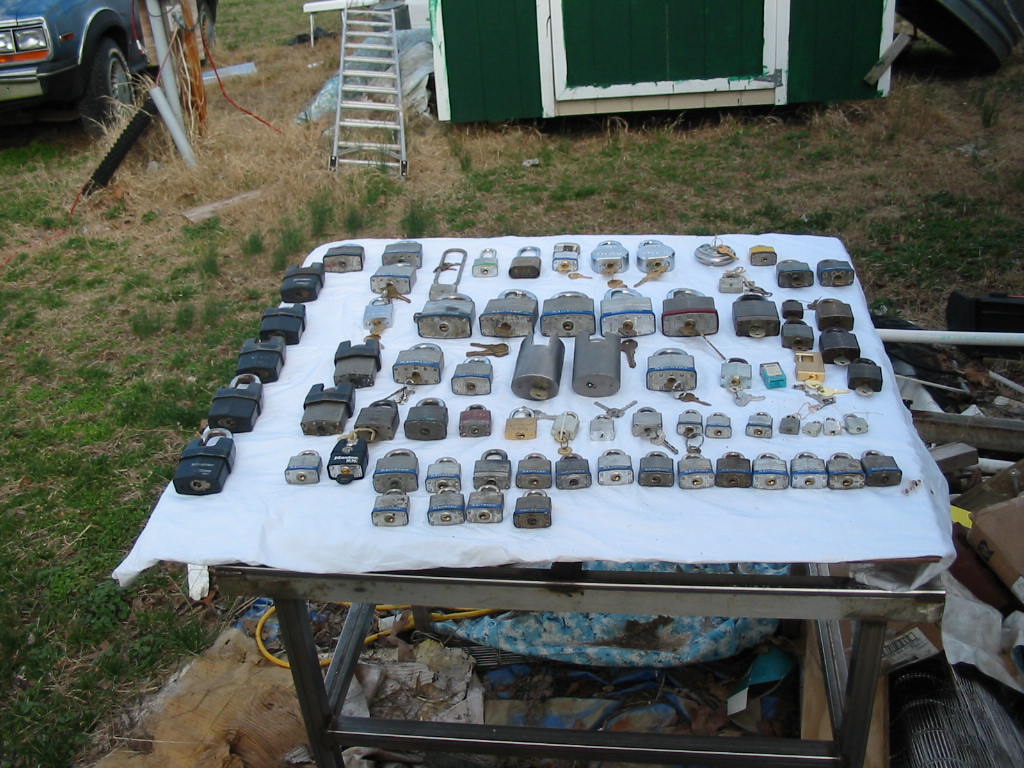The image depicts a scene outdoors featuring a makeshift metal table covered with a white cloth. Spread meticulously across the cloth are well over 50 padlocks of various sizes and colors. Most of the padlocks are either dark gray or light gray, with a few standing out in gold—one bright brassy gold and another in a subdued matte finish. Some padlocks have keys inserted, while others do not. They are uniformly arranged with the keyholes facing downward and the hasps upward, although the positions of the hasps vary, with only one being notably long. The surroundings include patchy green grass interspersed with straw, piles of miscellaneous junk, and the base of a green shed with white trim. A ladder rests nearby, and in the upper left corner of the image, the front quarter panel and wheels of a blue pickup truck are visible. This peculiar assortment of padlocks might suggest a testing setup or perhaps a collection obtained through magnet fishing.